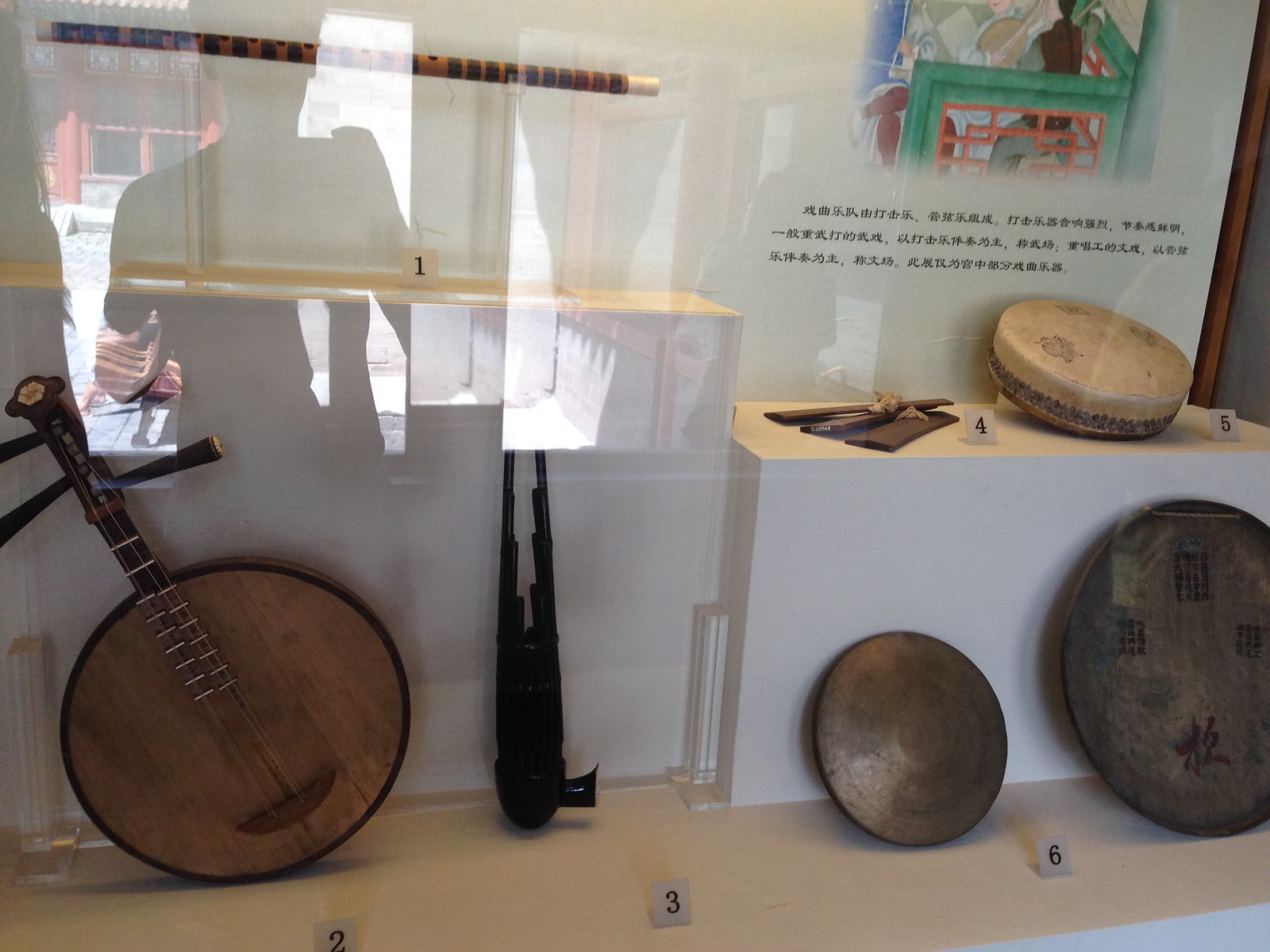The image showcases a meticulously arranged museum display of traditional Asian instruments and objects, all encased behind glass that causes some reflections. Central to the exhibit and numbered '2' is a round, guitar-like stringed instrument made from light brown wood, with a darker wooden neck strung with strings. To its right, numbered '6', is a small, circular, bronze cymbal. Left of the guitar is an object labeled '3', which appears to be a dark black item. Above these, on a wooden shelf, there is an ancient wood flute with a light and dark brown pattern, marked with '1'. Below it, numbered '4', are three flat brown blocks topped with cloth. Nearby, identified as '5', sits a tan drum with dark brown stitching made from hide. Also visible is another circular wooden item with Japanese writing, part of a mural that features green and orange hues and a fence with lettering in an Asian script. Each object is meticulously labeled, and the arrangement provides a fascinating glimpse into traditional musical instruments and items from Japanese culture, expertly curated in a museum setting.